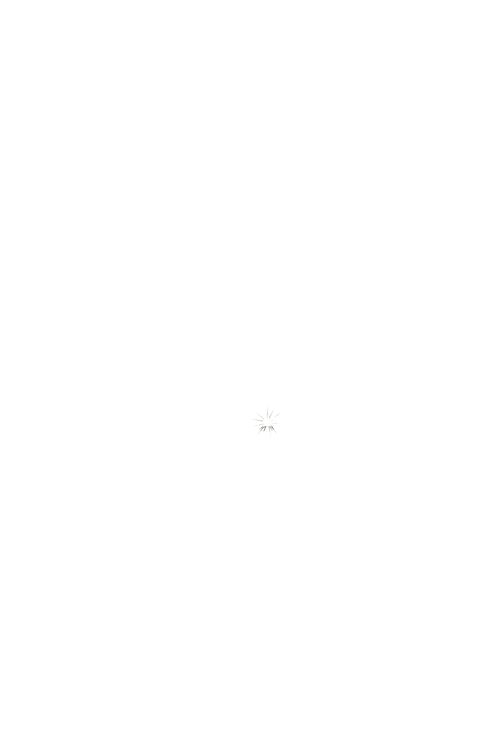Upon refreshing the page twice, I encountered an unusual image consisting solely of a small, star-like icon situated near the bottom of an otherwise entirely white background. The icon, approximately the size of a dime, features a white circular center with gray lines radiating outward, reminiscent of a tiny starburst or a windshield crack. Despite repeated attempts to reload the page, this peculiar icon consistently appears, slightly larger than the mouse cursor. This element could possibly be an informational or symbolic icon from a website, but no other elements or content accompany it on the screen.